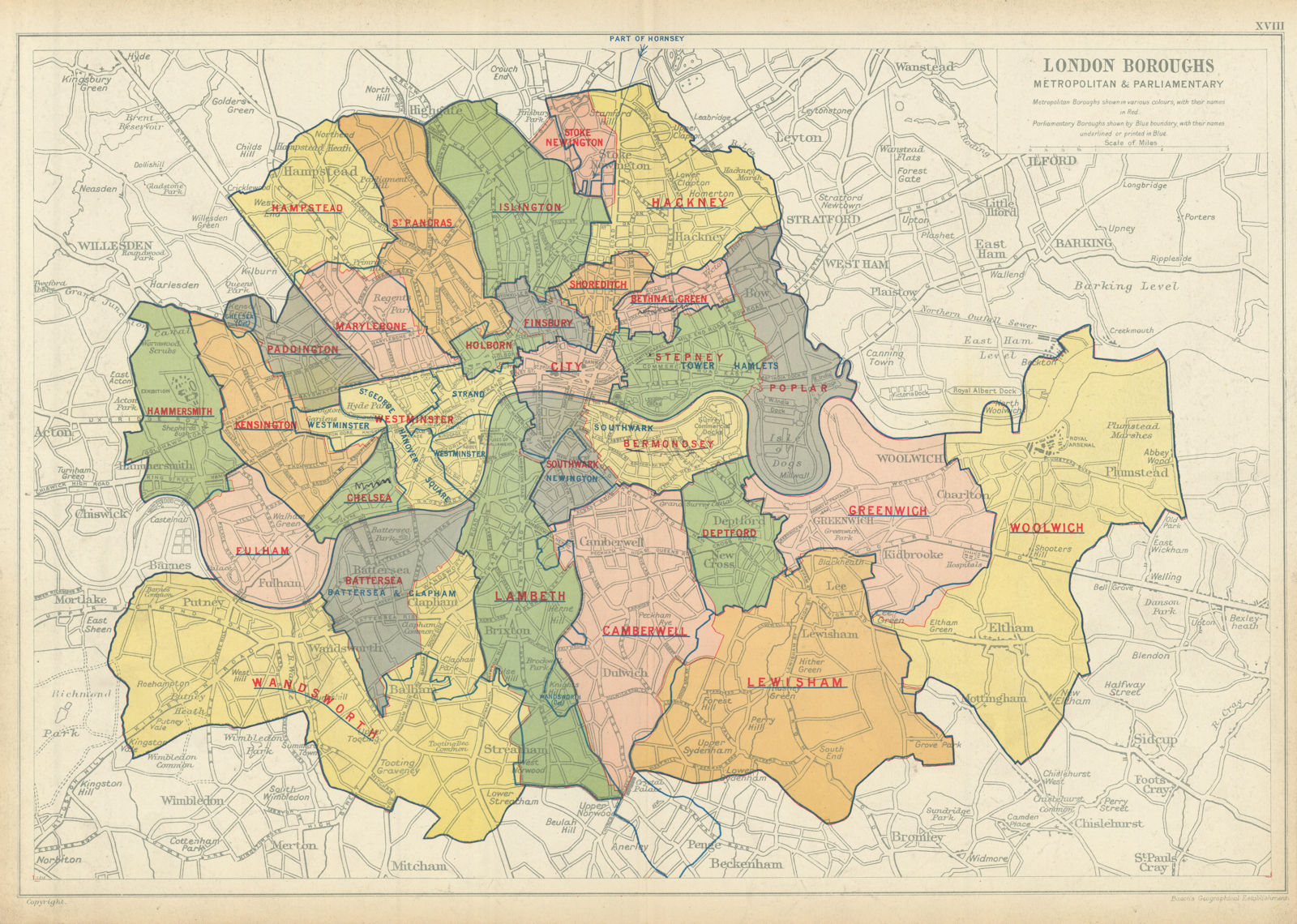This image features a faded, old-school map of London, prominently labeled at the top with "London Boroughs Metropolitan and Parliamentary." The map distinctly outlines various boroughs of London, using different shades—including green, orange, yellow, and gray—to demarcate boundaries. Notable boroughs such as Greenwich, Woolwich, Camberwell, Lambeth, and Wandsworth are clearly labeled in red lettering. The surrounding land, depicted in a more monochrome palette, adds contrast to the highlighted boroughs. The map appears to be quite dated, possibly from the 19th century, and lies flat, presenting a historical layout that may have evolved over time.